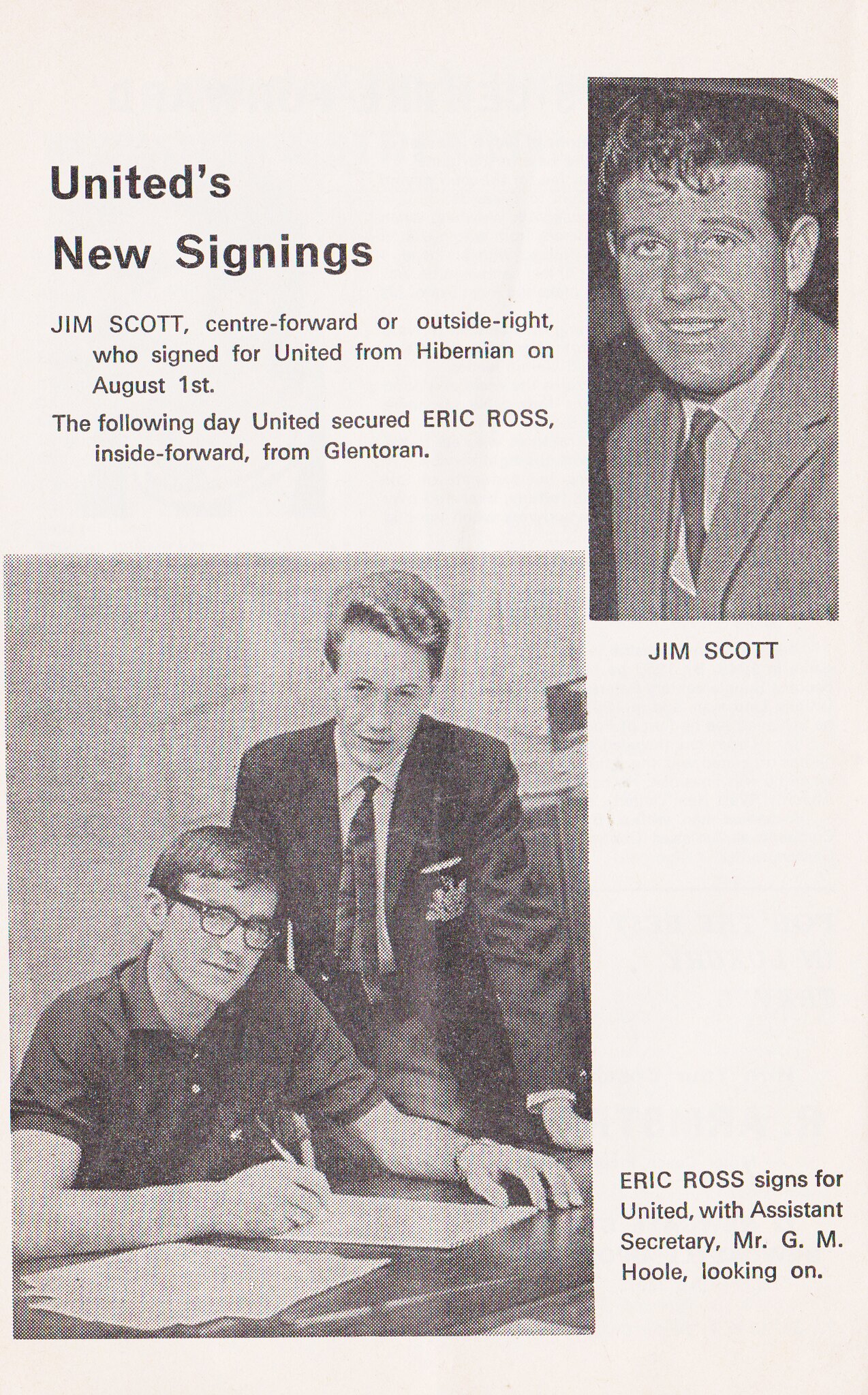The image is a page from a vintage magazine or newspaper, characterized by its tan, aged color. The page features two black-and-white photographs: one on the top right and one on the bottom left. In the top left corner, black text reads "United's new signings." Below this header is a detailed caption: "Jim Scott, center forward or outside right, who signed for United from Hibernian on August 1st. The following day, United secured Eric Ross, inside forward from Glentoran."

The photograph on the top right shows a man in a suit and tie, smiling, with a caption below identifying him as Jim Scott. The photograph on the bottom left features two men in the midst of signing a document, with one seated and the other standing, observing the process. To the right of this photograph, another caption in black text reads, "Eric Ross signs for United with Assistant Secretary Mr. G.M. Hull looking on."

These two images and descriptive texts together highlight the recent signings of players Jim Scott and Eric Ross by United, capturing a moment in the club's recruitment history.